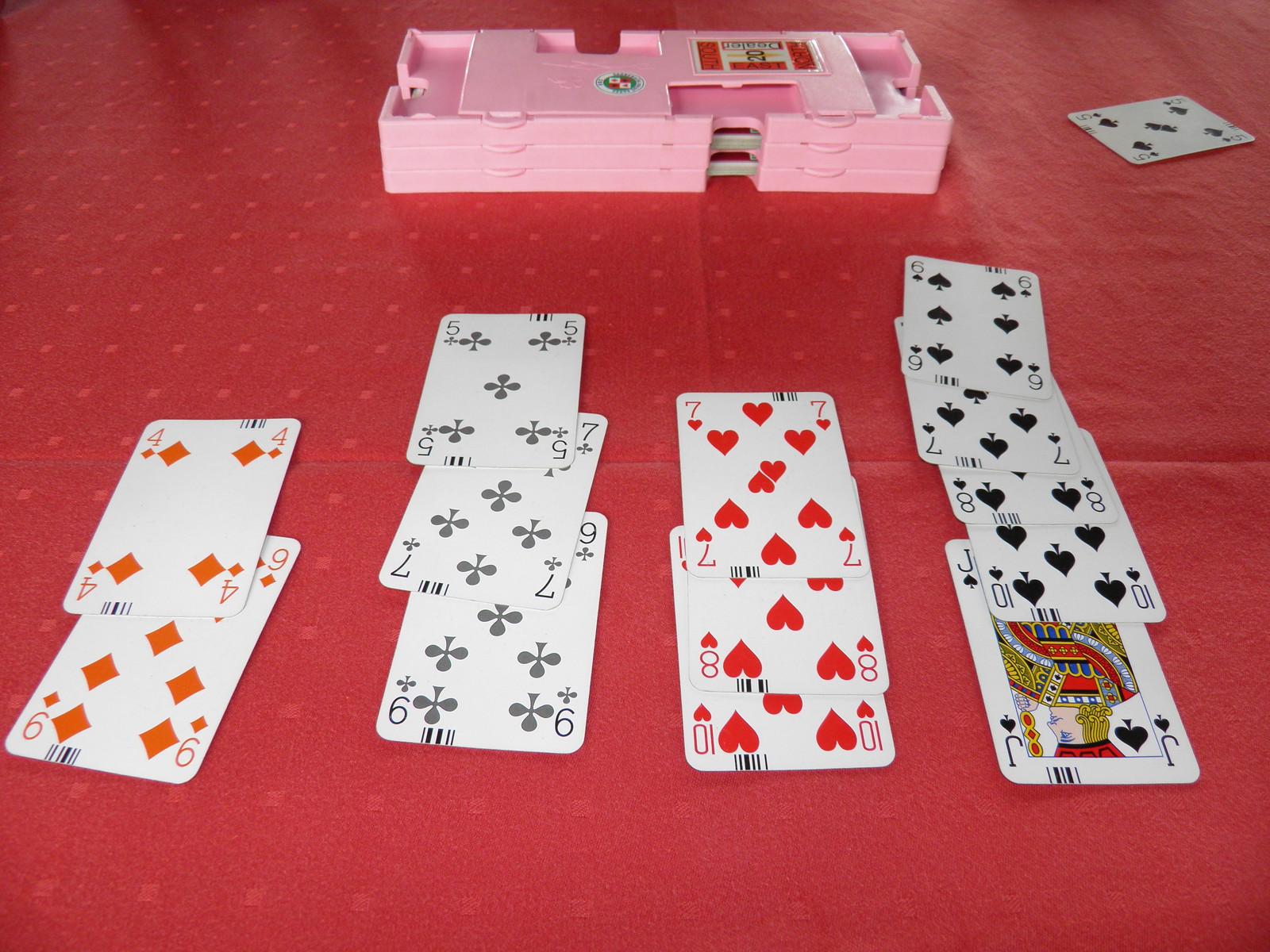The image depicts an organized arrangement of playing cards set on a red tablecloth, divided into four vertical rows, each representing a different suit. Here’s a detailed breakdown of the image:

- **First Row (Far Left)**: Two cards, both from the suit of diamonds. They are the Four of Diamonds and the Nine of Diamonds.
- **Second Row (Middle Left)**: Three cards, all clubs. These are the Five of Clubs, the Seven of Clubs, and the Nine of Clubs.
- **Third Row (Middle Right)**: Three cards, all hearts. These cards are the Seven of Hearts, the Eight of Hearts, and the Ten of Hearts.
- **Fourth Row (Far Right)**: Five cards, all spades. The cards are the Six of Spades, the Seven of Spades, the Eight of Spades, the Ten of Spades, and the Jack of Spades.

Additional details include a Five of Clubs card placed in the upper right-hand corner of the image. Moreover, there are four pink-colored plastic pieces stacked on top of each other situated in the upper middle section of the image.